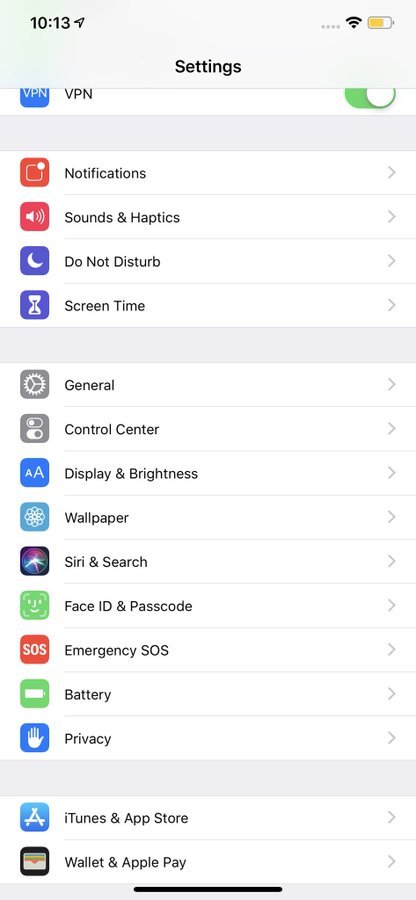This is a detailed screenshot of a smartphone's settings menu. The background color is predominantly white, with a very light blue-gray header at the top. On the left side of the header, the time is displayed as 10:13. On the right side, there is a gold battery icon indicating that the battery is approximately three-quarters charged, alongside a Wi-Fi icon that suggests a strong signal.

In the center of the header, the word "Settings" is prominently displayed. Below the header, the background remains white. On the left side, there is a comprehensive list of setting categories, each written in a medium-gray font with a corresponding icon on the left. The first grouping includes items such as Notifications, Sounds & Haptics, Do Not Disturb, and Screen Time, separated by a gray divider.

The list then continues with another set of categories: General, Control Center, Display & Brightness, Wallpaper, Siri & Search, Face ID & Passcodes, Emergency SOS, Battery, Privacy, and, at the very bottom, iTunes & App Store and Wallet & Apple Pay.